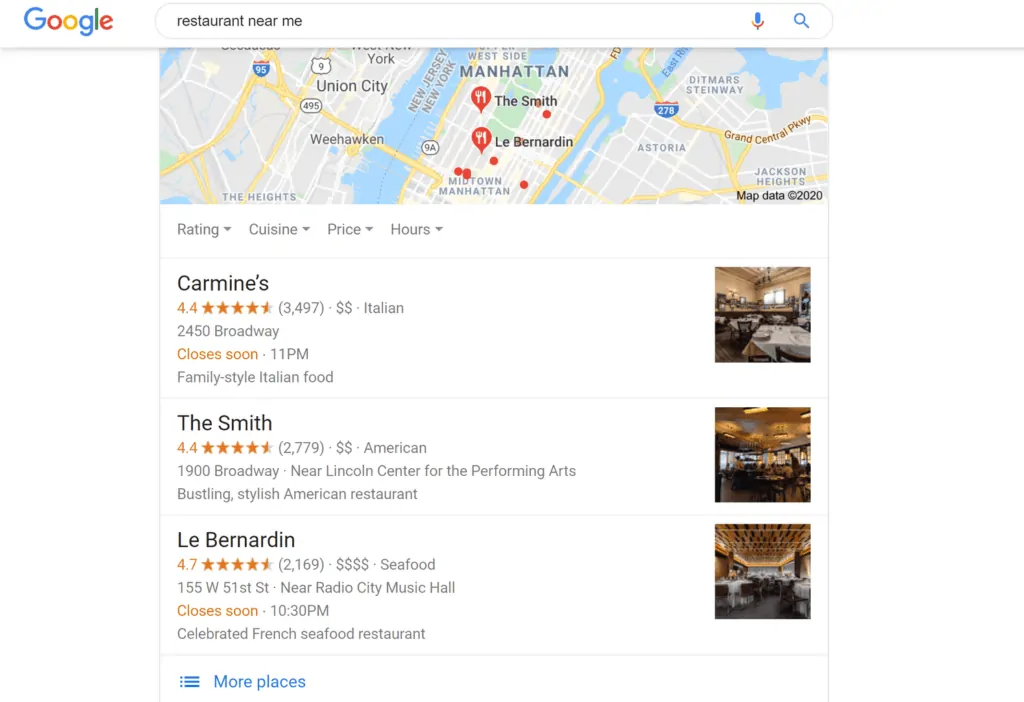The image depicts a screenshot of the Google website interface, highlighting a search query for "restaurant near me." In the upper left corner, the distinctive Google logo is visible, featuring its iconic blue, red, yellow, and green colors. The search bar prominently displays the query, complete with a microphone icon and the search button.

Below the search bar, a map of Manhattan, New York is shown. Two prominent red pins, each marked with a fork and knife, indicate specific food locations. Several additional red pins are scattered across the map.

Underneath the map, categories for sorting the search results are visible: Rating, Cuisine, Price, and Hours. Three restaurant listings are highlighted:

1. **Carmine’s**: This family-style Italian restaurant has a rating of 4.4 stars from 3,497 reviews. The rating and the note "Closes soon" are displayed in orange. The address is also listed, and a photo of the restaurant appears on the right side.
  
2. **The Smith**: An American cuisine restaurant, also rated at 4.4 stars based on 2,779 reviews. The rating is shown in orange, along with a photo of the restaurant's interior.

3. **Le Bernardin**: Specializing in seafood, this restaurant boasts a rating of 4.7 stars. Like the others, it features a corresponding photograph.

At the bottom of the listings, a link to "More places" is available in blue. Additionally, a menu bar for further search options is visible.